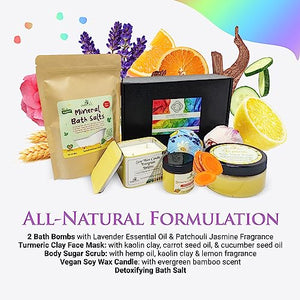This image is an advertisement for an all-natural formulation gift set comprised of various personal grooming and bath items. Dominating the scene are two bath bombs infused with lavender essential oil and patchouli jasmine fragrance, a turmeric clay face mask featuring kaolin clay, carrot seed oil, and cucumber seed oil, a body sugar scrub enriched with hemp oil, kaolin clay, and a lemon fragrance, as well as a vegan soy wax candle scented with evergreen bamboo, and a detoxifying bath salt. These items are meticulously arranged in jars, pouches, and a standing cardboard package with a mirror behind them. The backdrop is accentuated with illustrative elements of lemon slices, an orange slice, and leaves, possibly representing jasmine, creating a visually appealing and cohesive display. The advertisement emphasizes the "all-natural formulation" in both text and product composition, highlighting natural and beneficial ingredients such as kaolin clay, essential oils, and fragrances derived from flowers and fruits. The image also features elements like roses, lavender, cucumbers, and carrots in the background, reinforcing the natural and organic theme of the product set.